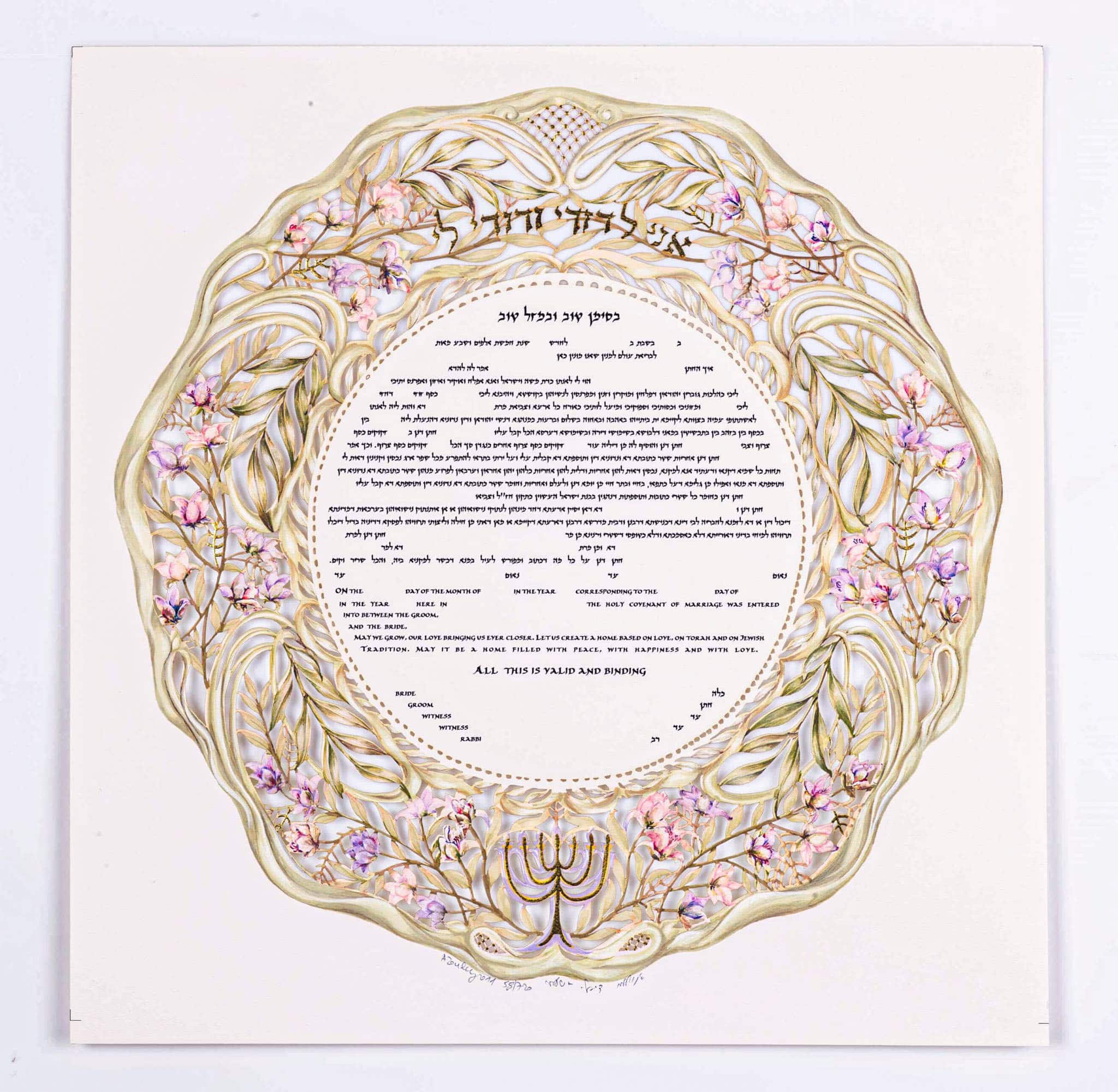This image depicts a highly ornate decorative plate embossed on square white paper, which rests on a white backdrop with a thin shadow adding depth. The plate features intricate golden spirals and floral decorations along its border, interspersed with sprigs bearing small, painted purple flowers. At the bottom of the plate, there is a black symbol resembling a seven-armed candle holder, possibly a menorah. The border encircles a central white area containing text in a non-Arabic script, likely Greek or Hebrew, with very small lined text in the same alphabet. The text at the top in black possibly indicates a title. Although the object’s exact nature (whether a painting, poem, or another type of artwork) is uncertain, its complex design and dual-use of gold and pink hues, along with black textual elements, emphasize its decorative and possibly cultural significance.